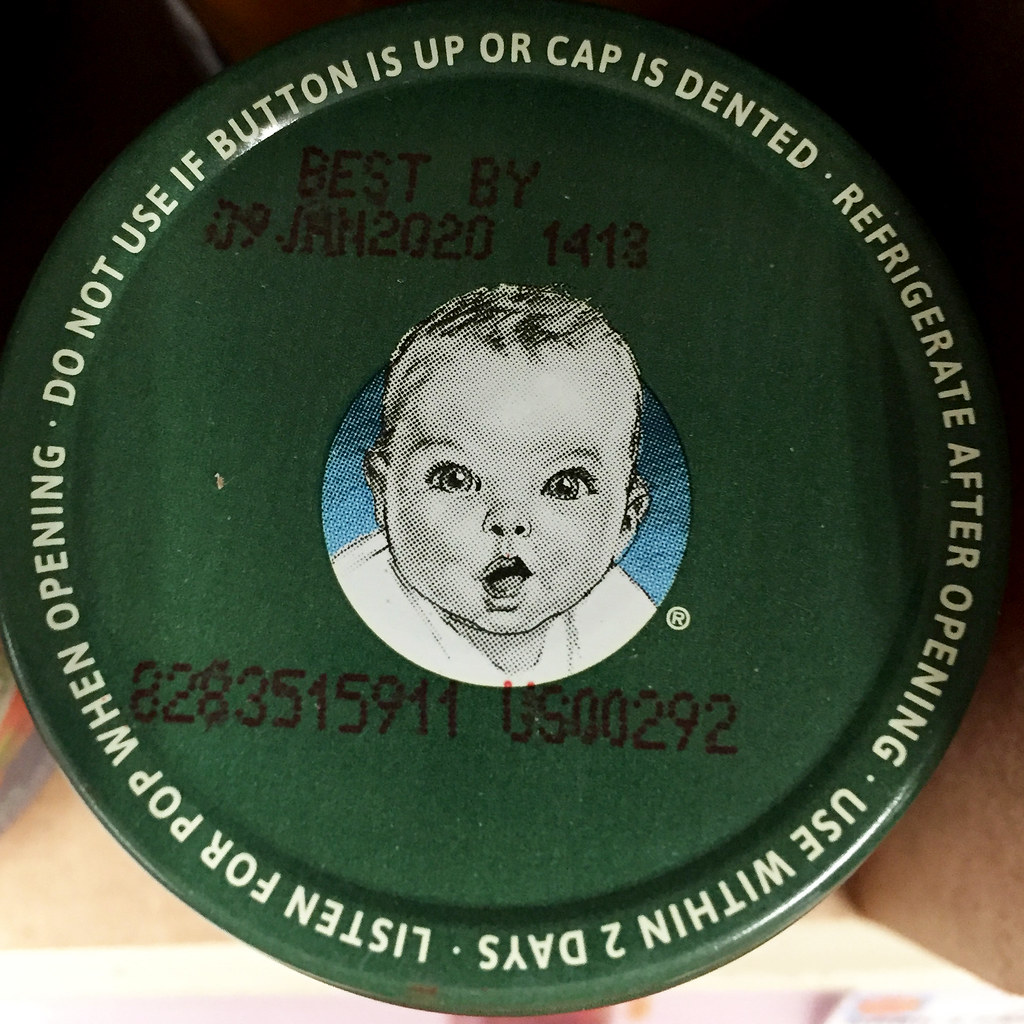This image captures the top view of a Gerber baby food jar's green cap. The cap is a dark green shade with a central illustration of the iconic Gerber baby. Encircling the edge in white lettering, there are various instructions, warnings, and details. It reads: "Do not use if button is up or cap is dented. Refrigerate after opening. Use within two days. Listen for pop when opening." Additionally, there is a "Best By" date of January 9, 2020, alongside a numerical sequence "1413." At the bottom of the cap, a code "8283515911 US 00292U" is printed.